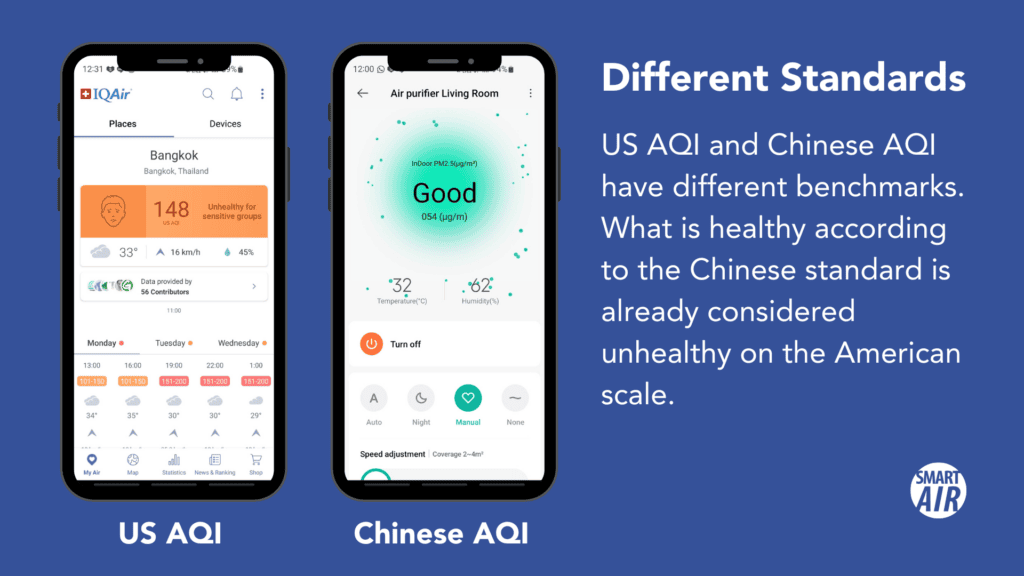The image showcases a page displaying detailed data comparisons between two smartphones placed side-by-side. The smartphones present contrasting Air Quality Indices (AQI) from the US and China, emphasizing their differing standards. According to the US AQI, a reading of 148, highlighted in orange, categorizes Bangkok, Thailand's air quality as "Unhealthy for Sensitive Groups." Conversely, the Chinese AQI, with different benchmarks, would view a similar reading as "Good." The smartphones also provide a comprehensive set of additional weather data, including temperature, precipitation percentage, and varying figures for air quality ranging from 101 to 200 over Monday, Tuesday, and Wednesday. Moreover, one screen displays further environmental details such as a temperature of 32°C and humidity at 62%, along with a 'turn off' button and various operational settings like auto, night, manual, or none. The page effectively highlights the variances in health standards for air quality between the two countries.